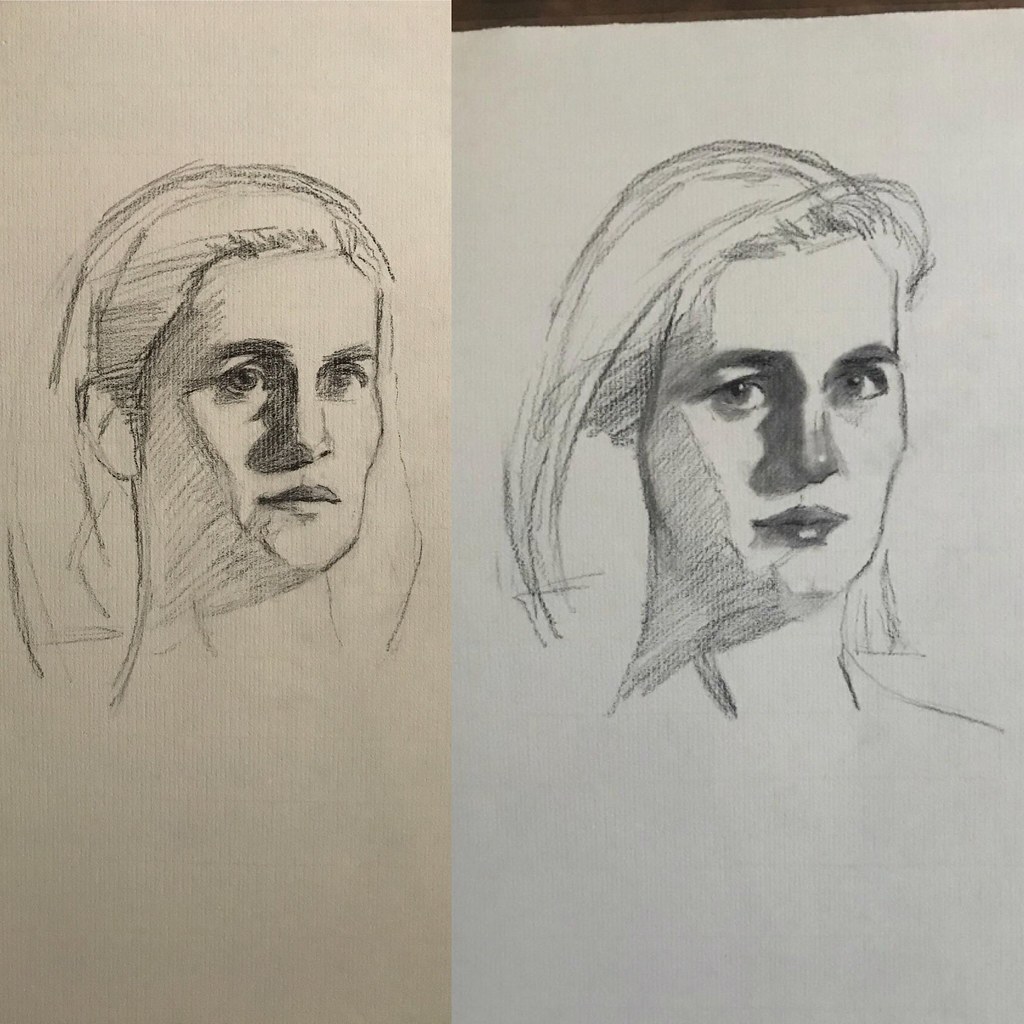The image features two pencil sketches of the same woman placed side by side on different colored papers: the one on the left is on a beige background and the one on the right is on a grayish-white background. Both drawings spotlight a woman with detailed facial features, but there are distinct differences in how these features are rendered and shaded.

The sketch on the left presents a woman with loosely drawn hair, lightly sketched eyebrows, large eyes, a defined nose, and thin, angled lips. The shading is subtle, giving a somewhat unfinished, minimalist impression. Her gaze appears distant, as though she's looking past the viewer. The facial expression communicates a sense of brooding or contemplation, and the overall drawing has a more raw and unpolished look.

In contrast, the drawing on the right portrays the same woman but with a more vivid and polished appearance. The hair is styled more deliberately, swept off to the side, and the eyebrows are thicker and better blended. The eyes are more lively and less scratchy, with more detail and depth. The nose is blended smoothly, and the lips are fuller and appear to have lipstick, giving them a pouty look. She seems to be looking directly at the viewer with a more assertive and engaging expression. Notably, the right-side sketch features some unfinished elements, like the faint outline of the hair and an undetailed ear, contributing to a sense that this version, while more vibrant, remains incomplete.